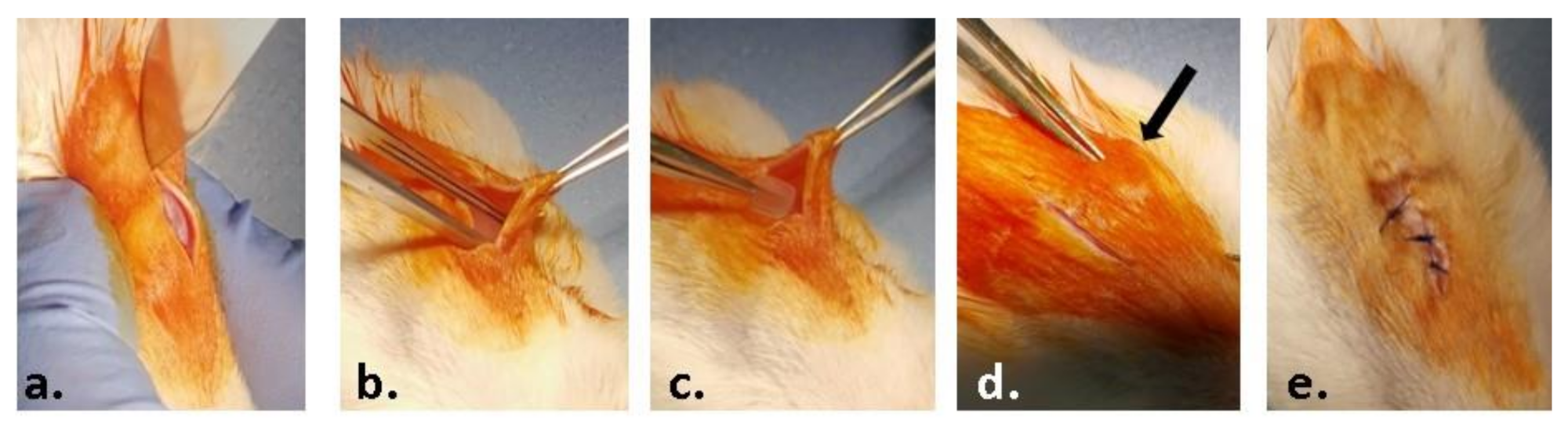The image is a series of five labeled photographs, A through E, depicting a veterinary surgical procedure on an animal with a brownish-orange leg and white fur, likely resting on a bluish fabric. In image A, a visible incision reveals the flesh beneath the fur. Image B shows two silver metallic tweezers, the first holding the skin open and the second inserted into the cut. In image C, the tweezers extract a small, clear, square-like object. Image D indicates the tweezers resting on the surgical site with a black arrow pointing to the area, while image E displays the incision sutured closed with black stitches. The progression covers the surgery from the initial cut to the successful extraction and final stitching.